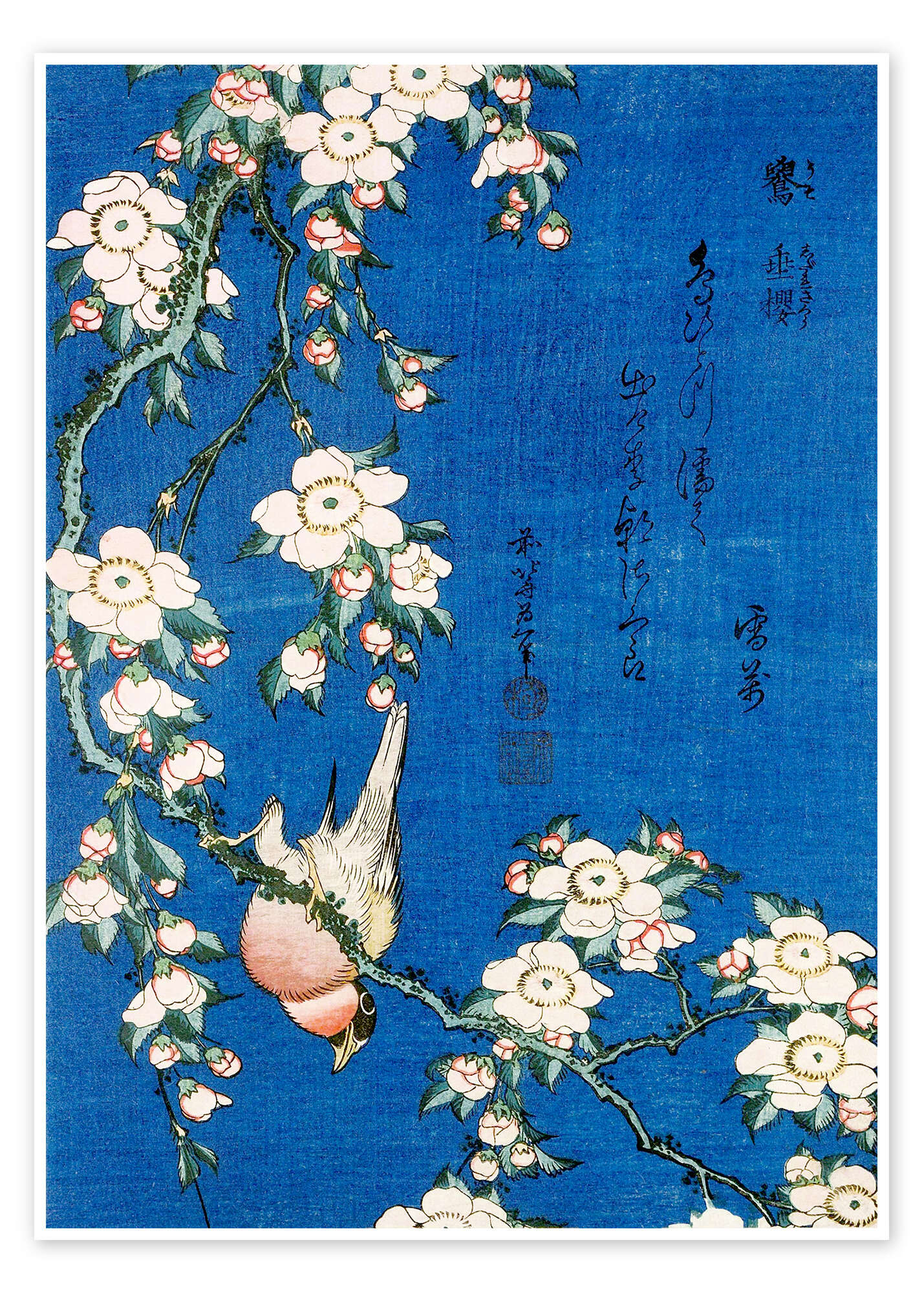This tall, rectangular image resembles a classic Japanese painting with a navy blue, hand-drawn background. At the center of this blue expanse, which shows hints of texture likely from colored pencils or similar mediums, runs a prominent vertical piece of black brushstroke writing. This writing extends from the top right towards the center of the image and concludes with two traditional stamp seals—one circular and one square—placed towards the bottom.

Spanning diagonally from the top left to the bottom right is a delicate tree branch adorned with numerous white cherry blossoms, each with yellow centers, as well as pink and white buds that haven't yet opened. Near the bottom left of the image, perched on the branch, is a small bird with striking colors: a black head, pink chin and belly, and a red body. The bird is uniquely positioned, standing upside down as it seems ready to peck at the flowers near it. The scene combines elements of both detailed natural beauty and traditional Japanese aesthetic influences, creating a vivid and enchanting artwork.